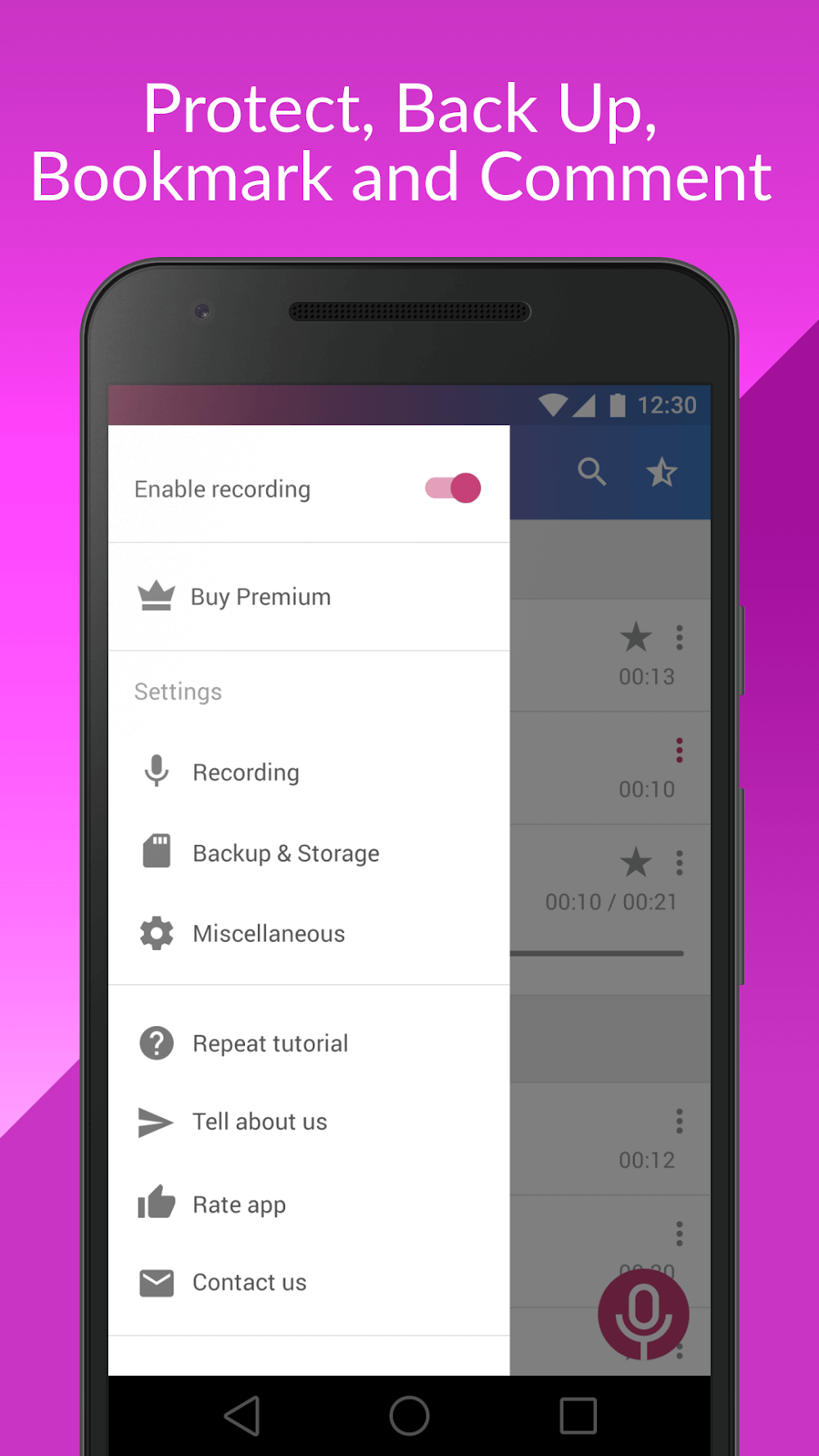Here's a detailed and cleaned-up caption for the image:

---

This vibrant advertisement showcases the impressive features of a smartphone on a split-screen background with an engaging diagonal transition from light to dark purple hues. At the pinnacle above the phone, the screen displays key functionalities labeled as "Protect," "Backup," "Bookmark," and "Comment."

The central focus is a detailed image of the phone, highlighting essential information like Wi-Fi connectivity and a 12% battery life indicator. The left sidebar of the image presents a navigational menu with options listed vertically. These options include:
- *Enable Recording* (selected)
- *Buy Premium* (accompanied by a crown icon)
- *Settings*
- *Recording, Backup and Storage*
- *Miscellaneous*
- *Repeat Tutorial*
- *Calabala, Great App*
- *Hot Tables*

Each menu item is complemented by intuitive icons: a microphone, a crown, a settings gear, a storage folder, a star, a question mark, an arrow, a thumbs-up, and an envelope respectively.

Adjacent to this menu, the main screen of the phone reveals partial recording timestamps due to the "Enable Recording" bar obstructing full visibility. Visible timestamps include segments of 13 seconds, 10 seconds, an incomplete 10 out of 21 seconds line, followed by a solid light gray box, and another 12-second segment. At the bottom, a distinctive red microphone icon signifies the recording function.

This image captures the intricate details and user interface elements, emphasizing the phone's recording and premium upgrade features.

---

This caption provides a thorough description, orienting the reader with the key elements and their functional details, which are visually available within the advertisement.